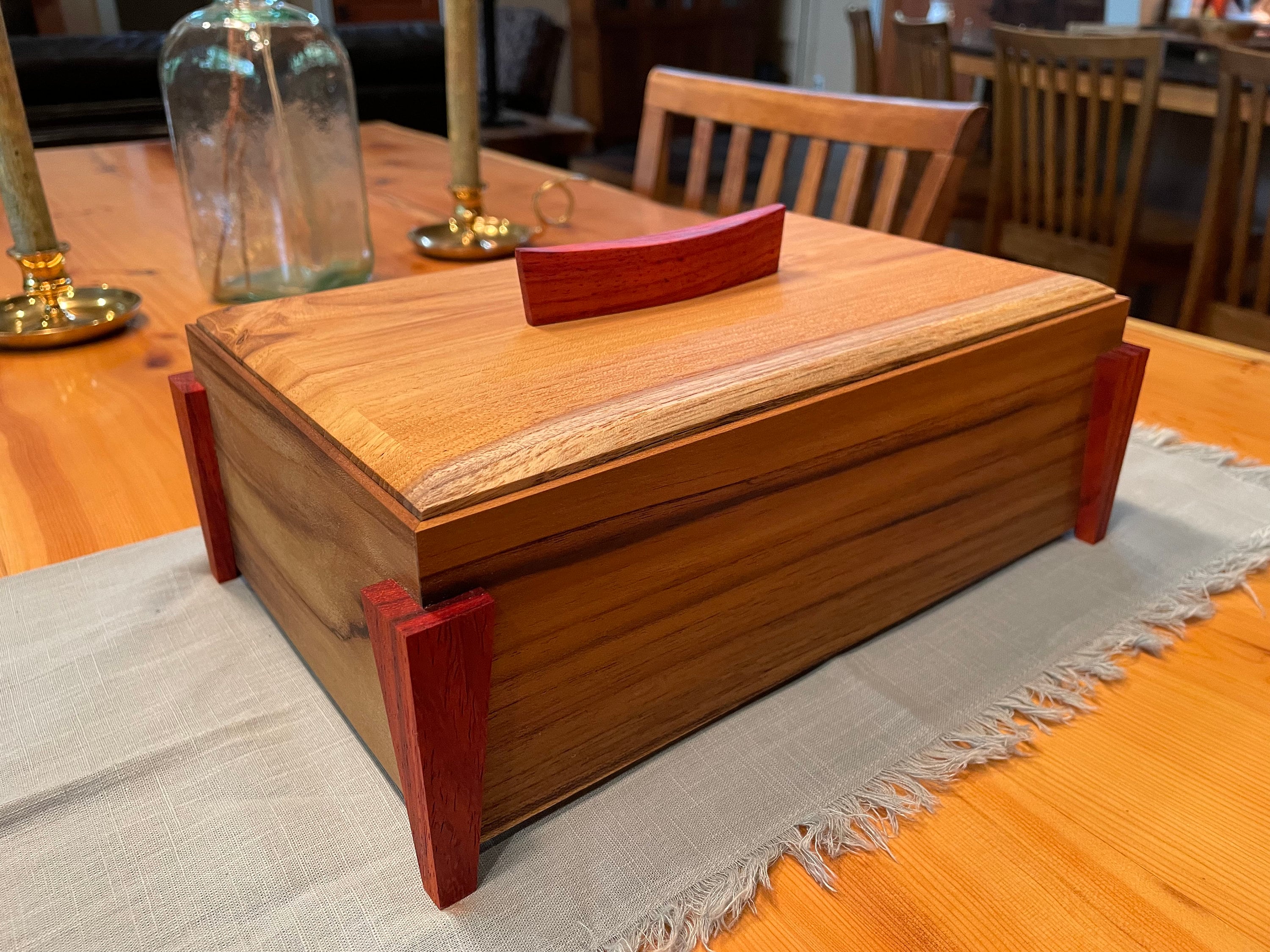The image showcases a detailed wooden box resting on an antique-style dining table, exuding an 18th-century charm. The box itself is small, approximately a foot long, nine inches wide, and six inches deep, constructed primarily from standard stained wood. It features a distinctive red wooden handle on the lid, with matching red wooden accents on the corners, possibly made of mahogany or cherry, while the main structure might be walnut. The box, with a simple finish and a lid that seems to lift off, is the focal point of the setting. The dining table, likely part of a restaurant or a space mimicking old-fashioned decor, is adorned with a glass bottle with a greenish hue, suggestive of being hand-blown, and two tall candles in holders. A placemat, sage green in color, further complements the rustic aesthetics. Additionally, a jar containing a dry floral arrangement sits in the center, enhancing the overall vintage atmosphere. The meticulous arrangement hints at a potential product image, possibly for a curated collection on an artisan platform like Etsy.